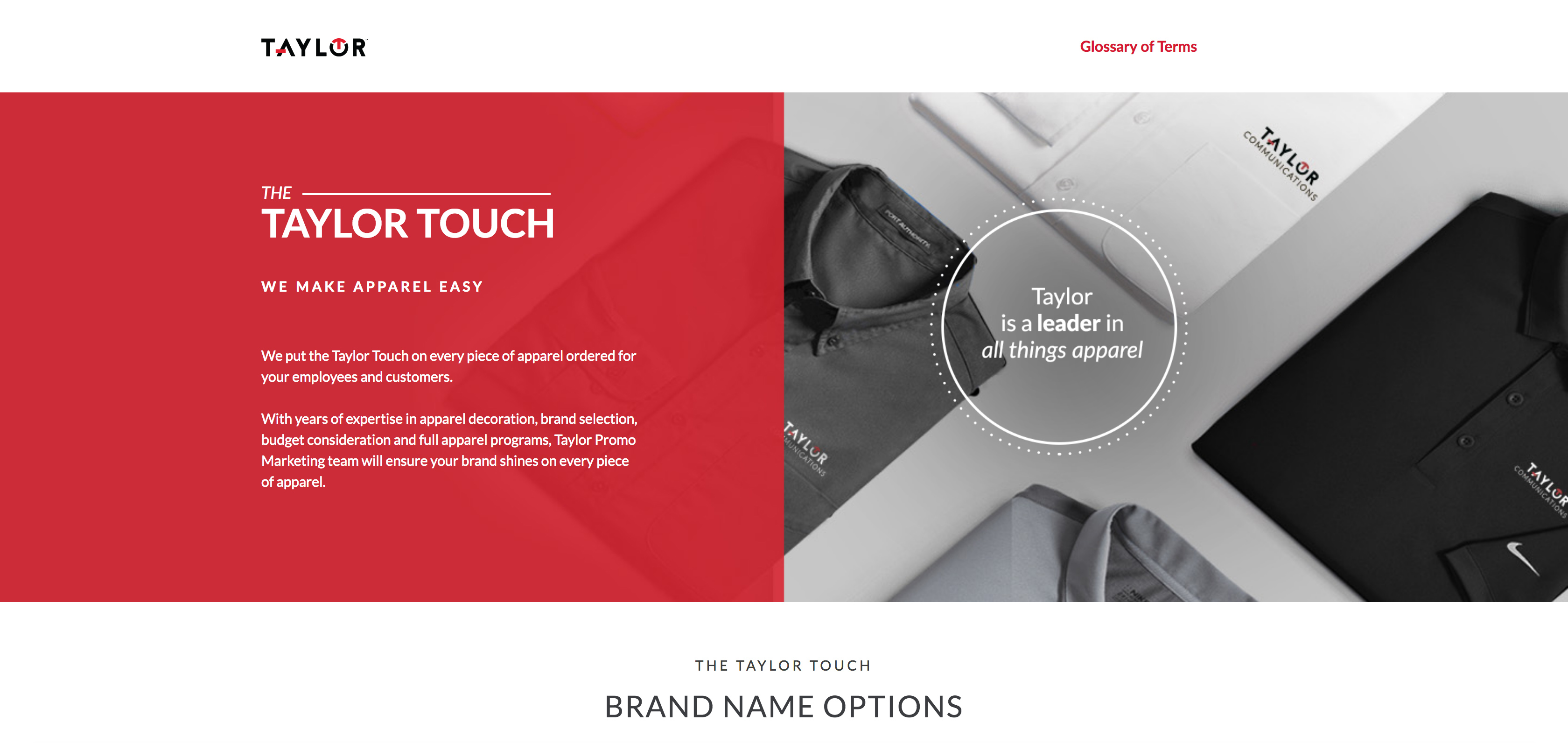The image features a professional website dedicated to a brand named Taylor. The site's header consists of a minimalistic design with a predominantly white background. On the left, the Taylor logo is prominently displayed, showcasing the word "Taylor" with stylish red accents. Adjacent to it is a red tab labeled "Glossary of Terms" in striking red text.

Beneath the header sits a bold red rectangle with white text that reads "The Taylor Touch." The accompanying slogan, "We make apparel easy," emphasizes Taylor's commitment to quality. Further text elaborates on the company's expertise: "We put the Taylor Touch on every piece of apparel ordered for your employees and customers. With years of expertise in apparel decorations, brand selection, budget consideration, and full apparel programs, Taylor's promo marketing team will ensure your brand shines on every piece of apparel."

To the right of this statement, the image showcases a series of folded polo shirts organized neatly in display cubbies. Although the image is in grayscale, the shirts appear to be in various colors including white and black. Superimposed over this display is a white circle bordered with dots, bearing the statement: "Taylor is a leader in all things apparel."

At the bottom of the image, black text reads "The Taylor Touch brand name options," grounding the design in a professional yet approachable manner.